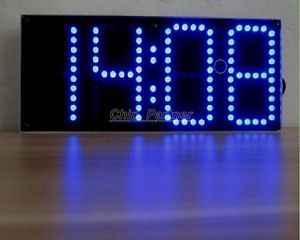This detailed caption describes an image of a small, rectangular, black bedside clock. The clock, which could be either a photograph or a design reference, takes up the upper half of the image, resting on a wooden table that occupies the lower half. The perspective is close-up, highlighting the simplicity and elegance of the clock. A knob on the right-hand side likely serves as a multi-functional control for the device. The clock displays the time "14:08" in neon blue dot-matrix numerals. Additionally, there appears to be a watermark, possibly reading "Chip Palmer" or "Chip Partner," overlaid on the image, hinting at either the designer or photographer's name.